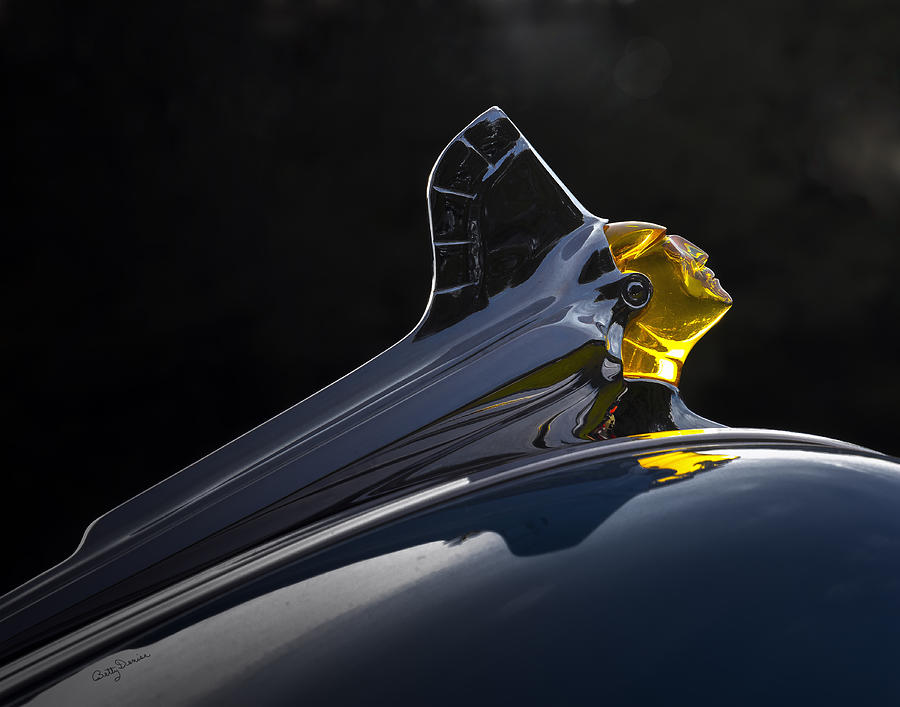The image displays a part of a 1952 Pontiac Catalina's hood ornament, prominently featuring a detailed chieftain head. Set against a pitch-black background that amplifies the reflective surfaces, the lower section of the image shows an oval-shaped, shiny black base. Extending from this base is a stylized metallic crest giving the impression of a headdress or mohawk, which is most elevated at the front before descending sharply as it extends backward. The centerpiece is a gold, illuminated depiction of a Native American chief. His face, viewed in profile, exhibits distinct Asian features with narrow, inset eyes, an aquiline yet flat nose, and a firmly set mouth. The chief's head is crowned by a crystalline yellow visage, which adds to the sense of illumination. The headdress has distinct lines at the top that blend into the background, accentuating the display's intricate design and craftsmanship.